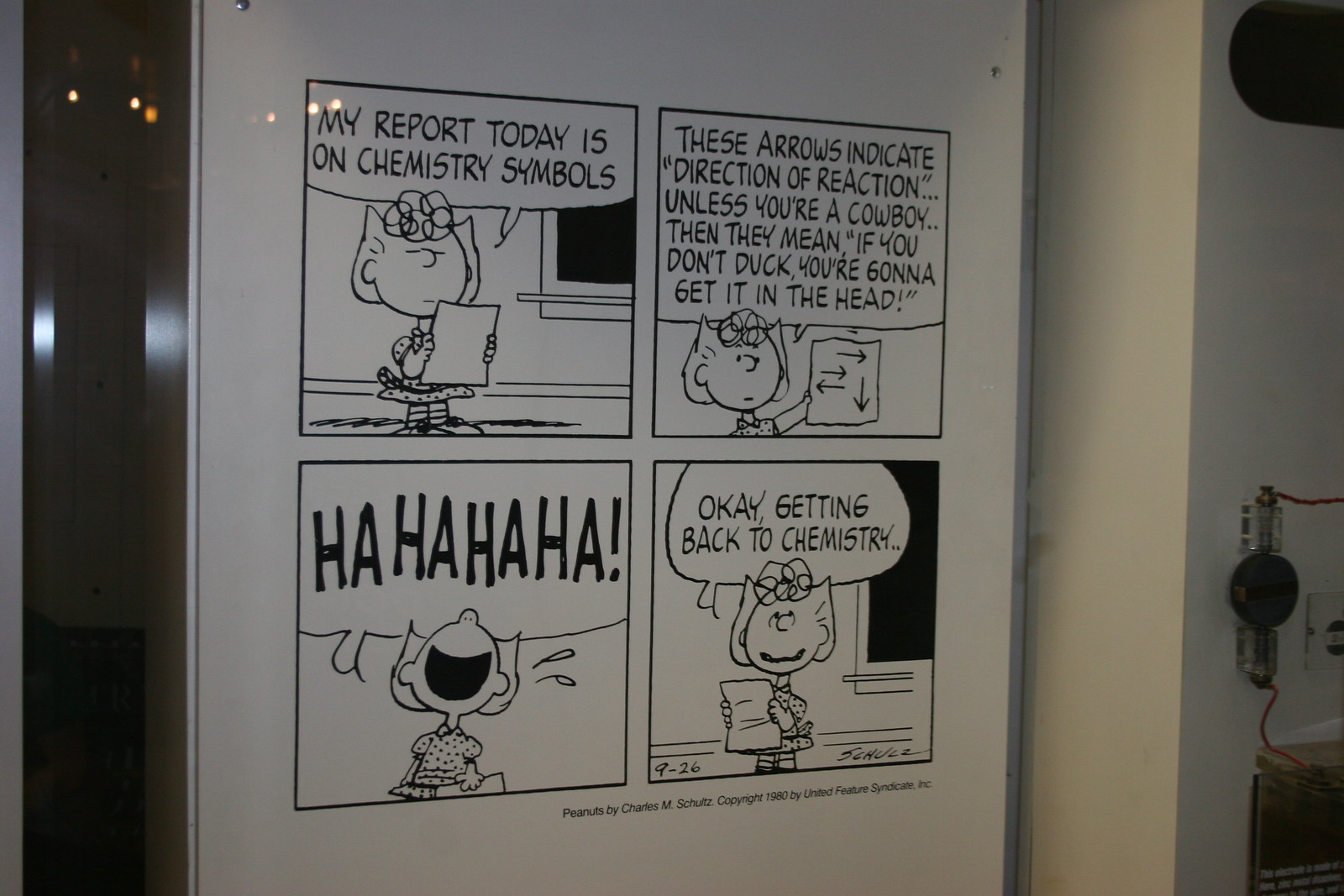Hanging on a beige-colored wall in the room, slightly visible on the far right, is a vibrant poster featuring a four-panel Peanuts cartoon. The comic strip stars Lucy, who is seen reading from a piece of paper in each panel. In the first panel, she confidently declares, "My report today is on chemistry symbols." In the second panel, she humorously explains, "These arrows indicate the direction of a reaction unless you are a cowboy. Then they mean if you don't duck you're gonna get it in the head." The third panel captures Lucy mid-laugh, her mouth wide open as she exclaims, "Ha ha ha!" Finally, in the fourth panel, Lucy resumes her composure, still holding the paper, and says, "Okay, getting back to chemistry." The poster adds a touch of whimsy and educational humor to the room, emphasizing Lucy’s comedic interruption during her presentation.